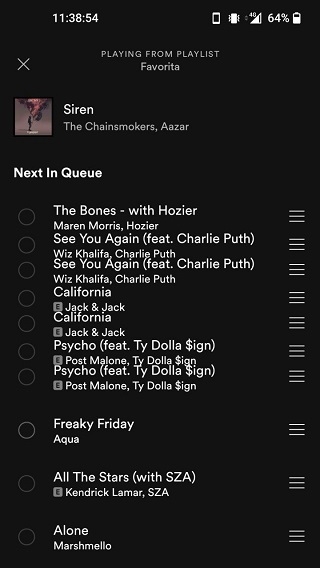Certainly! Here is a cleaned-up and detailed caption for the described image:

---

This image, captured on an iPhone screen, displays a music playlist interface. The notification bar at the top indicates a battery level of 64% and good signal strength, with the precise time shown as 11:38:54 AM. 

The screen features the music player from a playlist named "Favorite," though there's a slight typographical error in the title that reads "Favourite." The layout has a black background for a sleek, modern look.

On the left side of the screen, there's a small "X" icon, presumably for closing or exiting the playlist. The main section showcases the song "Siren" by The Chainsmokers & Aazar, along with what appears to be their album cover art.

Beneath this, the heading "Next in Queue" lists upcoming tracks:
1. "Bones" by Hozier
2. "California" by Jack & Jack (repeated twice)
3. "Psycho" featuring Ty Dolla $ign by Post Malone
4. "Freaky Friday" by Aqua
5. "All The Stars" featuring SZA by Kendrick Lamar
6. "Alone" by Marshmallow

Every element is clearly delineated, contributing to an organized and user-friendly display for navigating through the playlist.